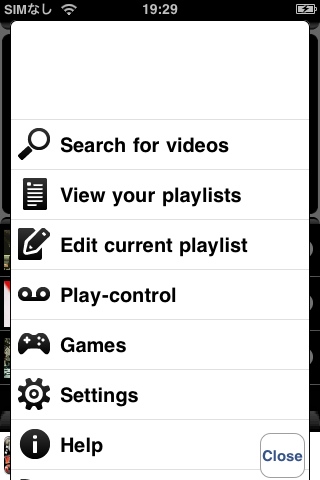Screenshot of a mobile phone displaying a detailed pop-up menu within an app or function. 

At the top, there is a black banner featuring various status icons: 
- On the top left, a SIM card icon accompanied by Asian writing symbols. 
- A fully serviced Wi-Fi symbol.
- In the center, the time displayed is 19:29.
- A fully charged battery icon with a lightning bolt indicating it is charging.

Below the black banner, the pop-up menu is set against a white background, showing several options organized in a list format:
- A blank, larger white section at the top.
- The first bar shows an icon of a magnifying glass with the label "Search for videos."
- The second bar displays an icon of a black paper with writing on it, labeled "View your playlist."
- The third bar features a pencil and paper icon with the text "Edit current playlist."
- The fourth bar showcases a voicemail symbol with the label "Play control."
- The fifth bar includes an icon of a game controller, labeled "Games."
- The sixth bar is depicted with a cog icon and the text "Settings."
- The last visible bar shows an information icon, a black circle with a white eye in the middle, and labeled "Help."

In the bottom far right corner, there is a "Close" button highlighted with blue letters within a light gray outlined box.

In the background, faint images resembling phone screen icons are visible, suggesting that this white screen pop-up menu is an overlay within a particular app or function.